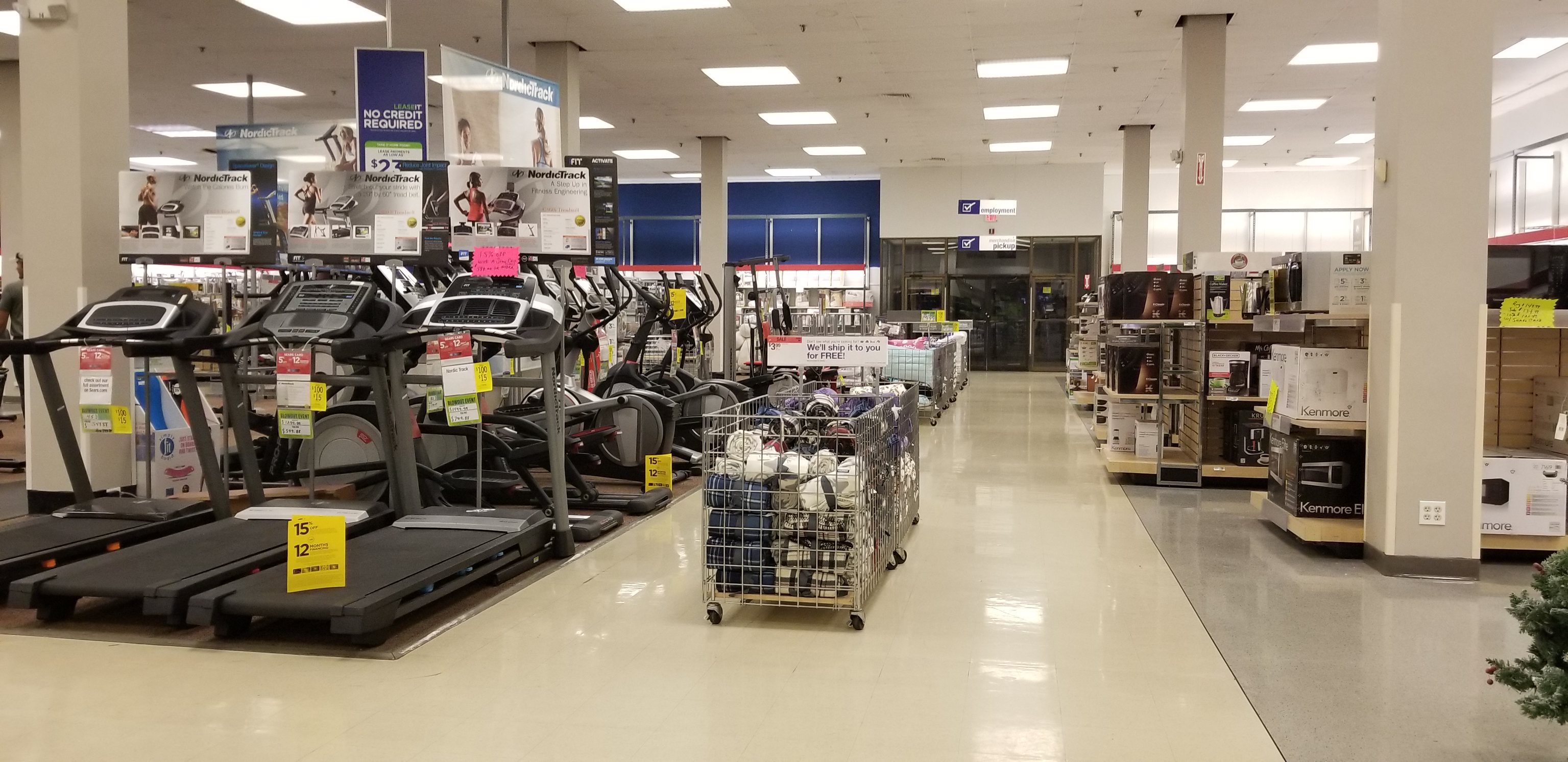This image captures a bustling department store, showcasing a variety of merchandise. On the left-hand side, there are shelves filled with assorted products for sale. In the center of the scene, three treadmills are prominently displayed. In front of the treadmills, a collection of bins is visible, each containing different items: one bin holds socks, another is filled with shoes, and a third appears to contain blankets, though their contents are somewhat indistinct. Various rows and aisles extend into the background, illustrating the extensive selection offered by the store.